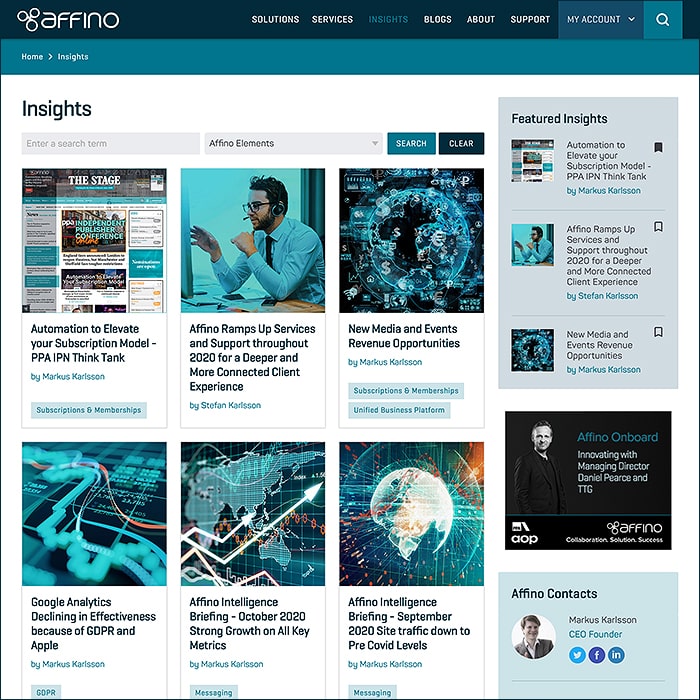A descriptive caption for the provided image could be:

---

Screenshot of Affino's website featuring a sleek and organized layout with a black header showcasing its logo—a triplet of white-bordered circles arranged in a triangular pattern, against a black rectangular background. To the right, the header lists navigation options in white all-caps text: SOLUTIONS, SERVICES, BLOGS, ABOUT, and SUPPORT, with INSIGHTS highlighted in blue. A smaller, dark blue rectangular box on the far right reads "MY ACCOUNT" with a dropdown arrow, accompanied by a teal square featuring a white-bordered magnifying glass icon. 

Below, the page transitions into a light gray border and a teal navigation bar with links to HOME and INSIGHTS, signified by white text and arrows. The main content area starts with the heading INSIGHTS in black, above a gray search bar labeled "ENTER A SEARCH TERM," and another search field pre-filled with "AFFINO ELEMENTS" next to SEARCH and CLEAR buttons.

The central section displays various publications and articles under INSIGHTS. Highlights include a publication titled "Automation to Evaluate Your Subscription Model, PPA, IPN THINK TANK by Marcus Carlson" linked by a blue box referring to "Subscriptions and Memberships." An adjacent image shows a person at a desk with a headset, captioned “AFFINO RAMPS UP SERVICES AND SUPPORT THROUGHOUT 2020 FOR DEEPER AND MORE CONNECTED CLIENT EXPERIENCE BY STEVEN CARLSON."

Next, an article titled "NEW MEDIA AND EVENTS REVENUE OPPORTUNITIES BY MARCUS CARLSON" is displayed next to a visual representation portraying financial data within a surreal cellular setting, captioned "GOOGLE ANALYTICS DECLINING IN EFFECTIVENESS BECAUSE OF GDPR IN APPLE BY MARCUS CARLSON."

Further below, a map underlines an international briefing "FINO INTELLIGENCE BRIEFING OCTOBER 2020 STRONG GROWTH ON ALL KEY METRICS BY MARCUS CARLSON," next to a globe projecting beams of light labeled “FINO INTELLIGENCE BRIEFING SEPTEMBER 2020 SITE TRAFFIC DOWN TO PRE-COVID LEVELS BY MARCUS CARLSON."

On the right, a sidebar displays featured insights in a smaller format, a black-and-white image labeled "AFFINO ONBOARD INNOVATING WITH MANAGING DIRECTOR DANIEL PEIRCE.” Beneath this, the logo and "Afino Collaboration Solutions Success” are highlighted, followed by contacts like a round image of a smiling man, Marcus Carlson, labeled CEO and Founder. The footer includes social media icons for Twitter, Facebook, and LinkedIn.

---

This detailed caption captures the intricate layout and specific elements present in the screenshot, providing a clear and comprehensive description of Affino’s website as depicted.